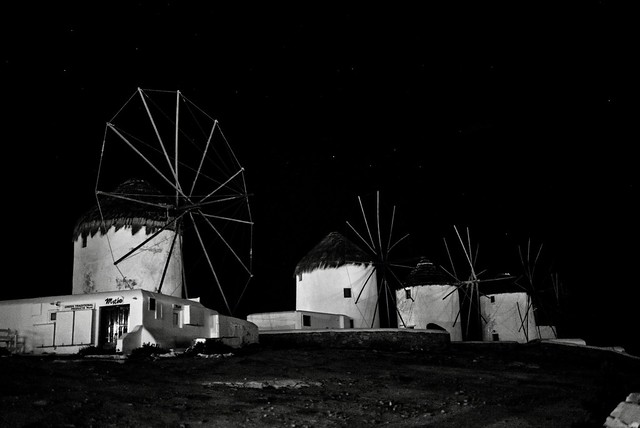A square black and white photograph taken outdoors at night features a dark, starless sky serving as the backdrop. Dominating the scene are four white cylindrical structures, most likely silos, each topped with a black, conical roof. These silos have small, blacked-out windows. In front of each silo stands a tall windmill, shaped like a wheel with spokes instead of traditional paddles, and appearing to be made of wood or metal. The ground is composed of dark, indistinct dirt and rocks, with what looks like a puddle slightly left of center. In the lower right corner, there's an undefined gray object. Surrounding the silos are shorter, one-story buildings with flat roofs, likely serving as auxiliary structures. The overall image is shrouded in nocturnal shadows, giving it a mysterious and somewhat eerie ambiance.